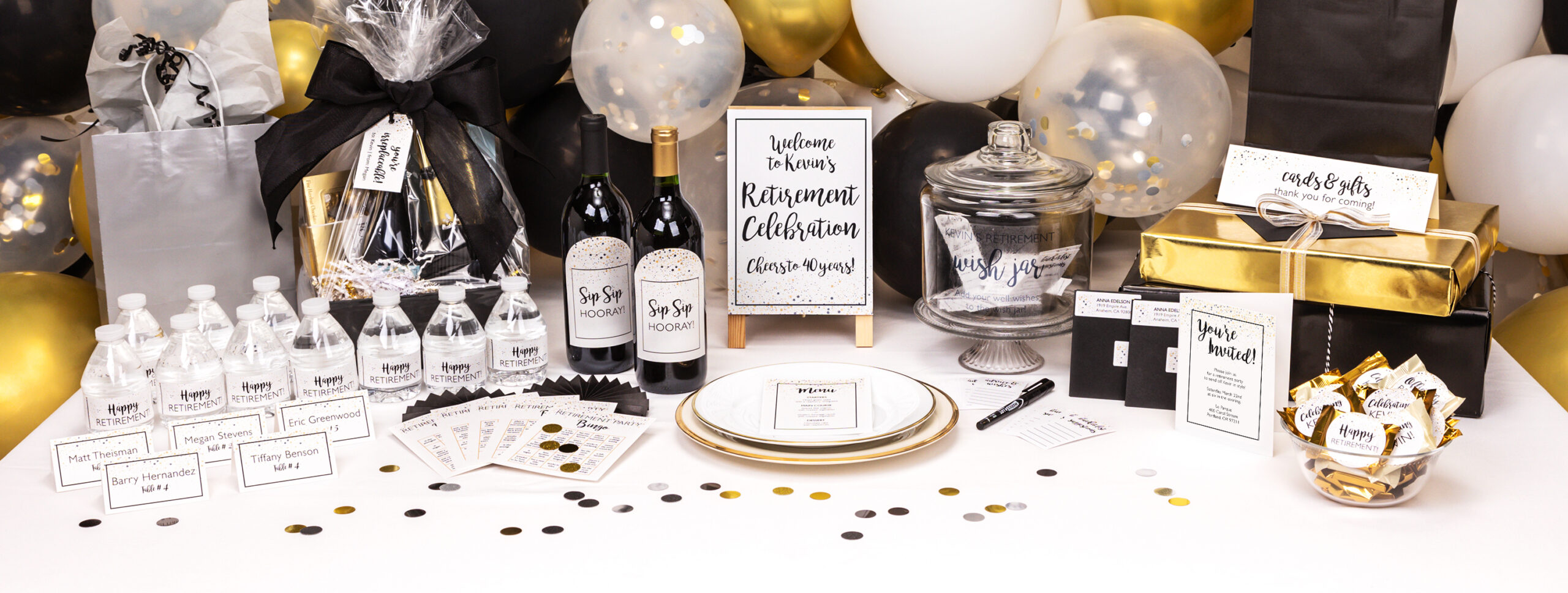This photograph captures a detailed table setting at Kevin's retirement celebration, emphasizing the theme of 40 years of service. Central to the display is a sign reading, "Welcome to Kevin's Retirement Celebration. Cheers to 40 years," printed in black script font on a white sheet with a black border, and adorned with silver and gold confetti dots at the bottom.

Arranged from left to right, the table features multiple items: on the far left, a cluster of small water bottles labeled "Happy Retirement," followed by neatly arranged name plates for guests, including Matt Theismann, Barry Hernandez, Megan Stevens, Tiffany Benson, and Eric Greenwood. A variety of festive elements enhances the scene, including gift bags and baskets wrapped in cellophane and tied with black bows, as well as gold, silver, and black balloons.

In the middle section, there's a glass jar labeled "Wish Jar," surrounded by papers and a sharpie for writing well-wishes. Notable is the presence of elegant white plates with gold rims, each holding a menu. Two champagne bottles, marked "Sip, Sip, Hooray," stand near the center—one features a black label, the other a gold one.

Closer to the right side, a bowl of candies inscribed with "Happy Retirement," and a box labeled "Cards and Gifts, Thank you for coming" sit alongside cards and a small invitation that reads, "You're Invited." This arrangement captures the celebratory atmosphere and detailed preparation for Kevin's milestone retirement event.